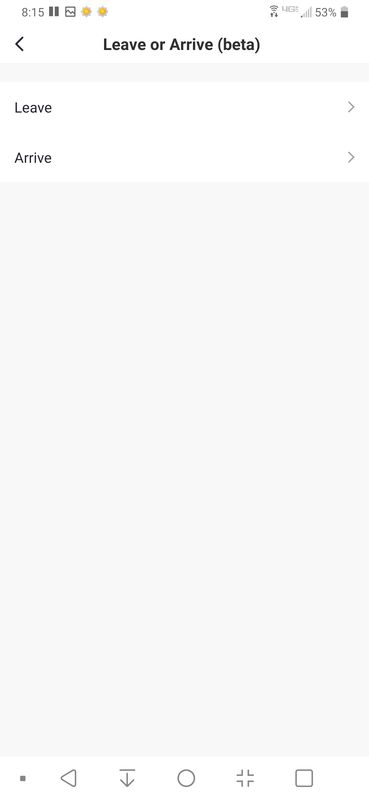This screenshot, captured from a smartphone, showcases the top section of the screen prominently displaying '8:15' in the upper left corner. Adjacent to this, on the upper right side, are several status indicators: two gray vertical bars, a square-shaped icon with a mountain-like figure in its center, and two yellow sun-like icons, suggesting various status notifications. In addition, the device shows connectivity icons including Wi-Fi, 4G, and four bars of cell reception, accompanied by a battery life indicator at 53%.

Centrally aligned below the status bar, the screen displays the text "Leave or Arrive (Beta)" with a left-pointing arrow situated to the far left. Beneath this text, there's a horizontal gray bar. Below this bar, on the left side, the options "Leave" and "Arrive" are listed on consecutive lines, each accompanied by right-pointing arrows at the far right of their respective lines. The remaining portion of the screen is largely dominated by an expansive, empty gray space, indicating a placeholder or yet-to-be-populated area of the app or webpage.